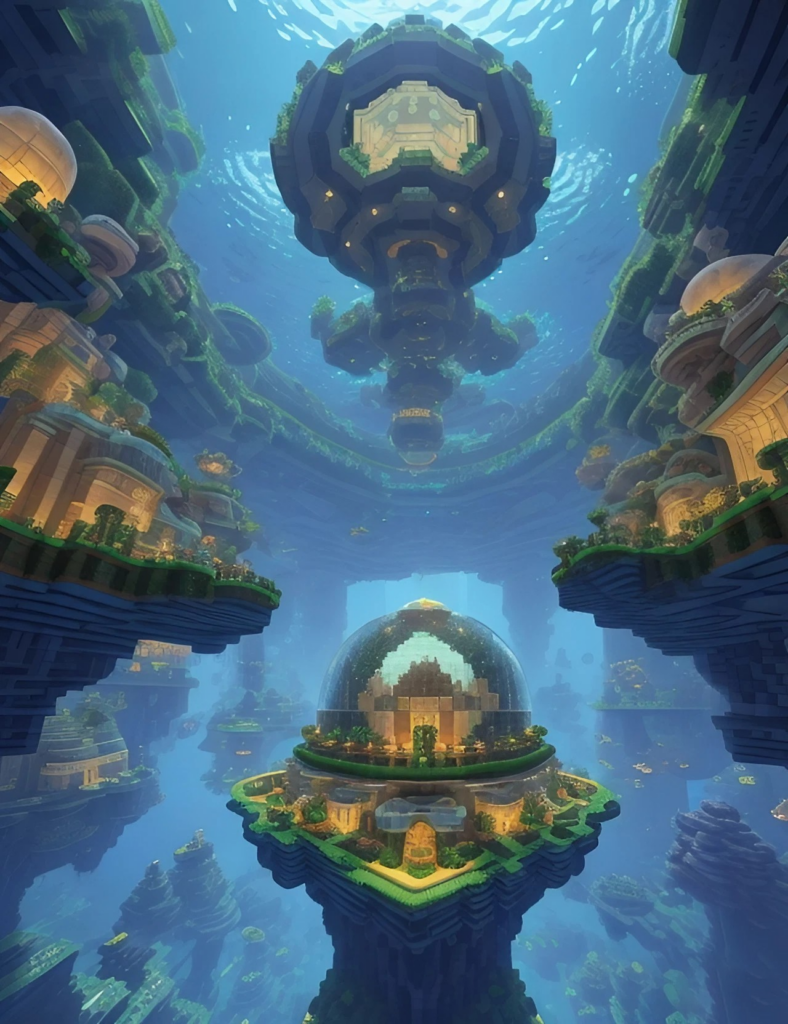This is a computer-generated image of an underwater city, reminiscent of a scene from a video game like Minecraft. The water is a light blue color with visible ripples at the surface. At the top, there’s a large, floating spherical structure, dark gray with yellow dots and green highlights, looking almost like a ball atop a stick-like base. This impressive structure casts a shadow over the underwater scene below.

Beneath this floating sphere, various underwater towers and plateaus are visible, each topped with arched domes that resemble glass. One prominent dome at the bottom encases something brown and is encircled by a green border, resting on a square platform adorned with yellow and green elements. These domes and platforms sit on rocky bases, creating an impression of stability. Surrounding the main structures, additional buildings are seen to the right and left, perched on rocky platforms, all shaded to amplify the underwater ambiance, highlighted in hues of green, brown, beige, and blue. The entire scene is illuminated by diffused light, enhancing the vibrant colors and illustrating the supposed underwater domain in detailed digital artistry.